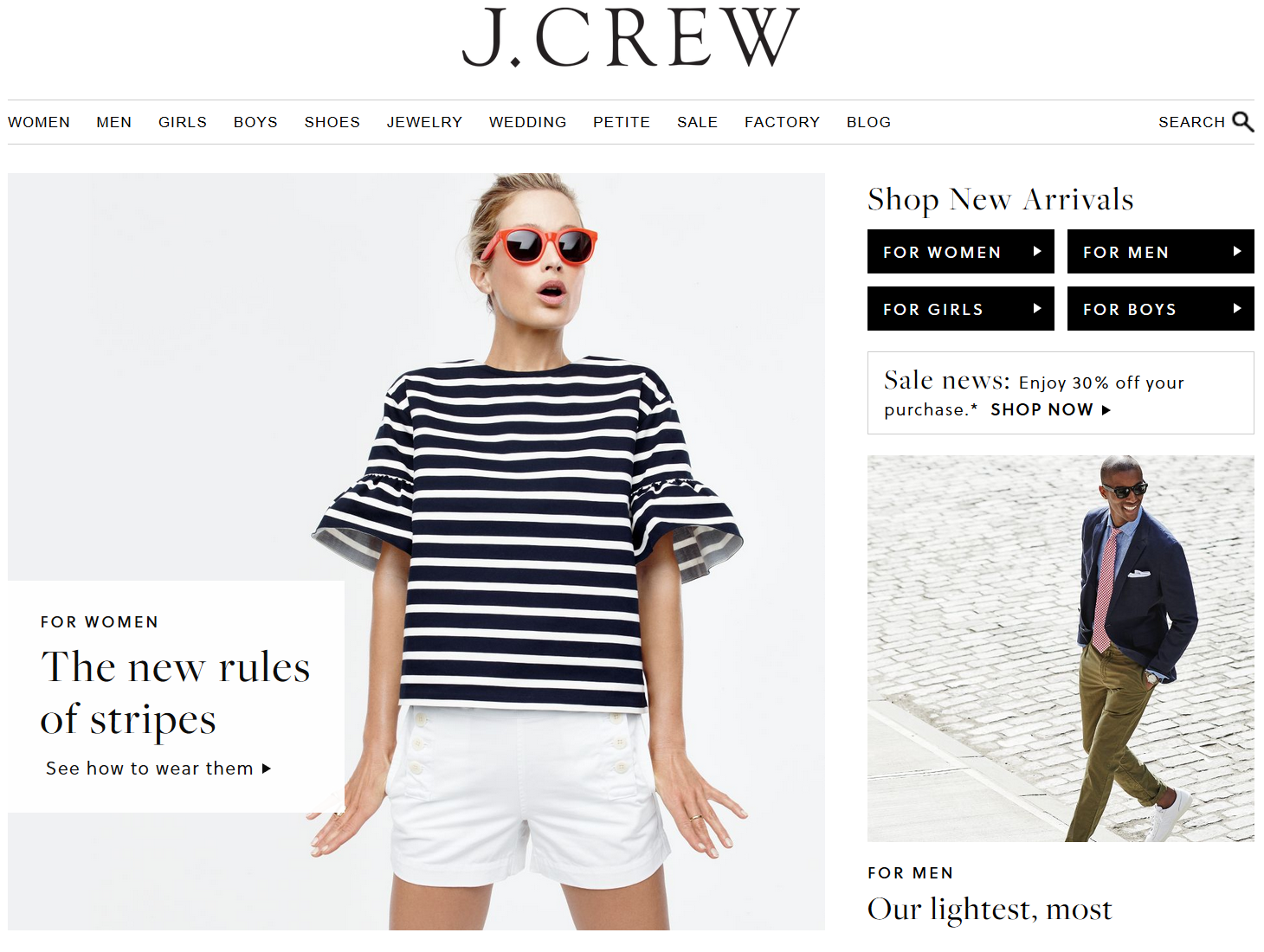On the homepage of J.Crew, we're presented with two photographs featuring models. 

The first image showcases a stylish female model, who is fair-skinned and sports playful orange sunglasses that resemble toy glasses, adding a quirky, hipster vibe to her appearance. Her hair is partially pulled back, and she is dressed in an off-the-shoulder top with horizontal black and white stripes. The sleeves of her top flare out near the elbows, further enhancing her chic look. She pairs her top with medium-length white shorts that are loose and gathered around the legs. The accompanying text reads: "For women: The new rules of stripes. See how to wear them."

The second image features a male model with striking black eyes, depicted in a casual walking pose through an urban setting. He exudes business casual elegance, dressed in a sophisticated blue blazer, brown khaki pants, and a pinkish-red tie. The caption near him reads: "For men: Our lightest, most..." before it cuts off. The website's interface prominently uses a black and white color scheme for its UI elements, emphasizing a modern and clean aesthetic.